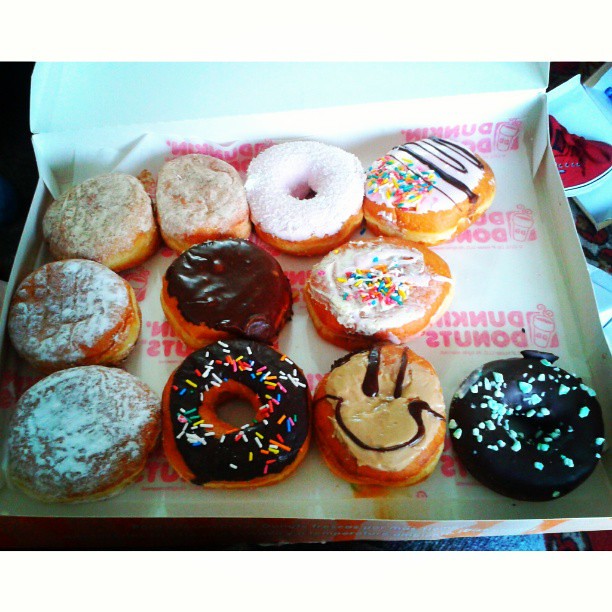This color photograph captures an open white donut box from Dunkin' Donuts, revealing an assortment of 11 donuts, with one missing from what would have been a dozen. The interior base of the box features an upside-down pastry tissue with backwards pink lettering that says "Dunkin' Donuts." The donuts are organized into three rows, with four in the top row, three in the middle, and four in the bottom row. The box holds a variety of donuts: there are powdered jelly donuts, cinnamon-topped jelly donuts, honey-glazed donuts with white frosting and chocolate swirls, and chocolate-covered donuts. One donut is adorned with multicolored sprinkles, while another features a peanut butter frosting with a chocolate drizzle smiley face. Additionally, there is a coconut donut with white frosting and a chocolate eclair. Positioned at the bottom right corner of the image, part of a person's knee clad in jeans can be seen, along with a glimpse of a red tennis shoe in the upper right corner, suggesting someone is holding the box on their lap.